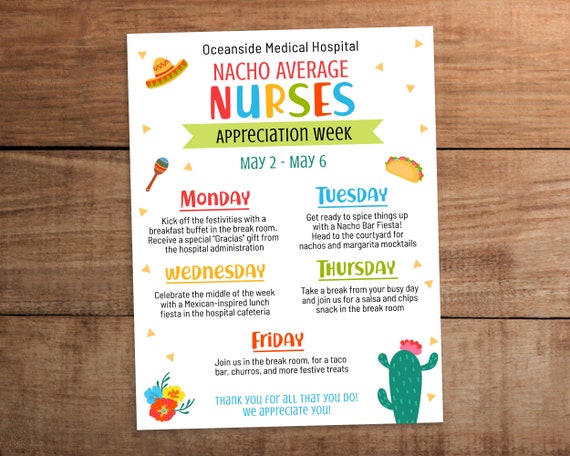The image depicts a vibrant and detailed flyer for "Nacho Average Nurses Appreciation Week," held by Oceanside Medical Hospital from May 2nd to May 6th. Set against a brown wooden background that resembles a table, the flyer is positioned on a white piece of paper and features colorful festive elements, including a green cactus with a pink flower, a fully loaded taco, maracas, a sombrero, and decorative flowers placed at the corners. Written in a combination of red and multicolored fonts, the flyer prominently displays its title and schedule, listing the daily festivities planned to honor the nurses. It concludes with a heartfelt message, "Thank you all for what you do. We appreciate you," emphasizing the appreciation for the nursing staff's hard work and dedication.